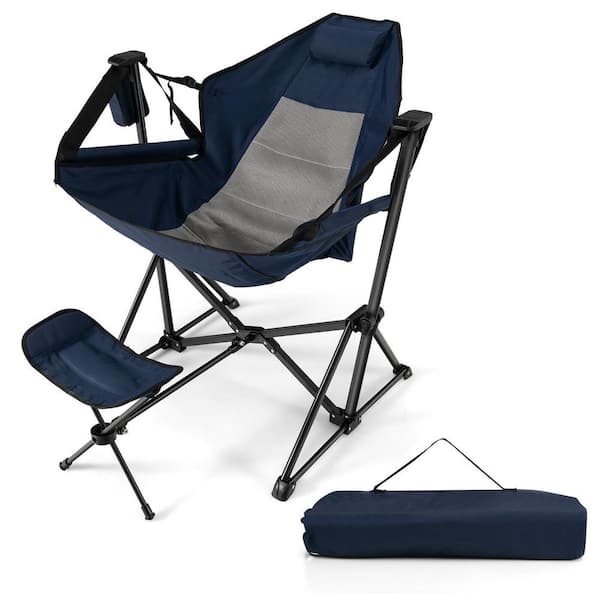This image showcases a navy blue fold-out camping chair set against a white background, centrally positioned and slightly to the left. The chair features a comfortable design with a deep, scooped seat and a built-in headrest. A distinct gray stripe runs down the middle of the chair's back and seat sections, further enhancing its aesthetic. The chair's sturdy frame is constructed from round black metal bars that extend to form a stable triangular base, with sliding clamps for easy collapsing and setup. 

On the right armrest, there is a practical cup holder for convenience. Extending from the front of the chair is a detachable footrest, made of the same navy blue fabric and supported by a black X-shaped metal frame, designed to lock securely into the chair to prevent tipping.

In the bottom right corner of the image, we see the chair's carry case, which is cylindrical in shape and made of the same navy blue material, complete with a black strap for shoulder carrying. This compact and durable case ensures easy transportation and storage, making the camping chair highly portable and ideal for outdoor activities.